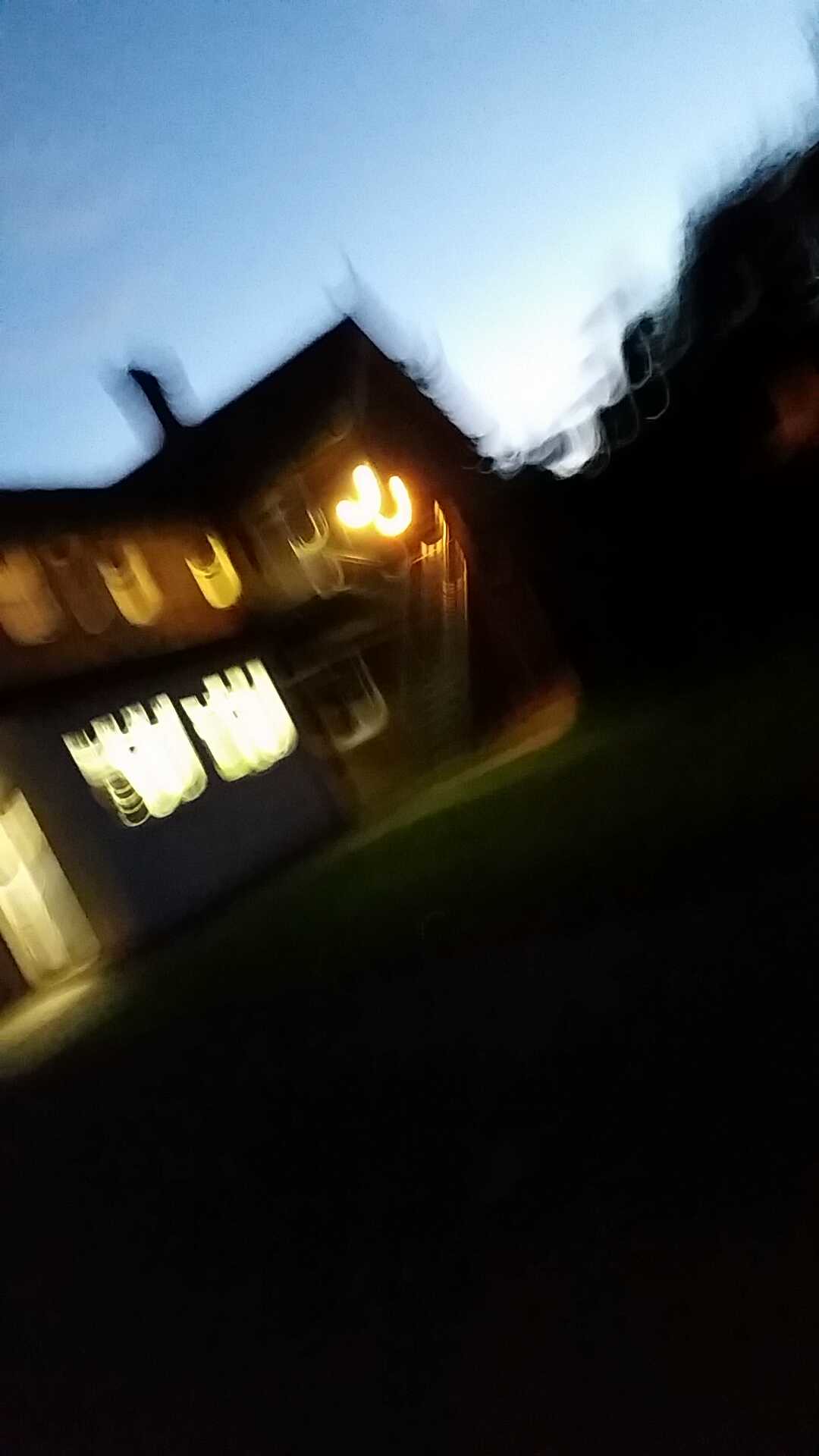This photograph, blurred and slightly distorted, captures an outdoor scene at twilight. Dominating the middle of the frame is a large, two-story house with a distinctive gable roof and a chimney. The house is illuminated, with several windows and a back door emitting a combination of bright white and warm orange light. The house, though blurry, reveals as many as seven windows, contrasting against the dark surroundings.

The sky above is a fading blue, indicating the sun has already set, casting a twilight glow over the scene. On the right side of the image, the silhouettes of trees are faintly visible. The lower half of the photo is enveloped in darkness, suggesting the photographer was standing in a dimly lit area, perhaps a lawn or yard, with grass just discernible through the gloom. This combination of twilight sky, illuminated house, and surrounding darkness creates a striking, if fuzzy, night-time snapshot.